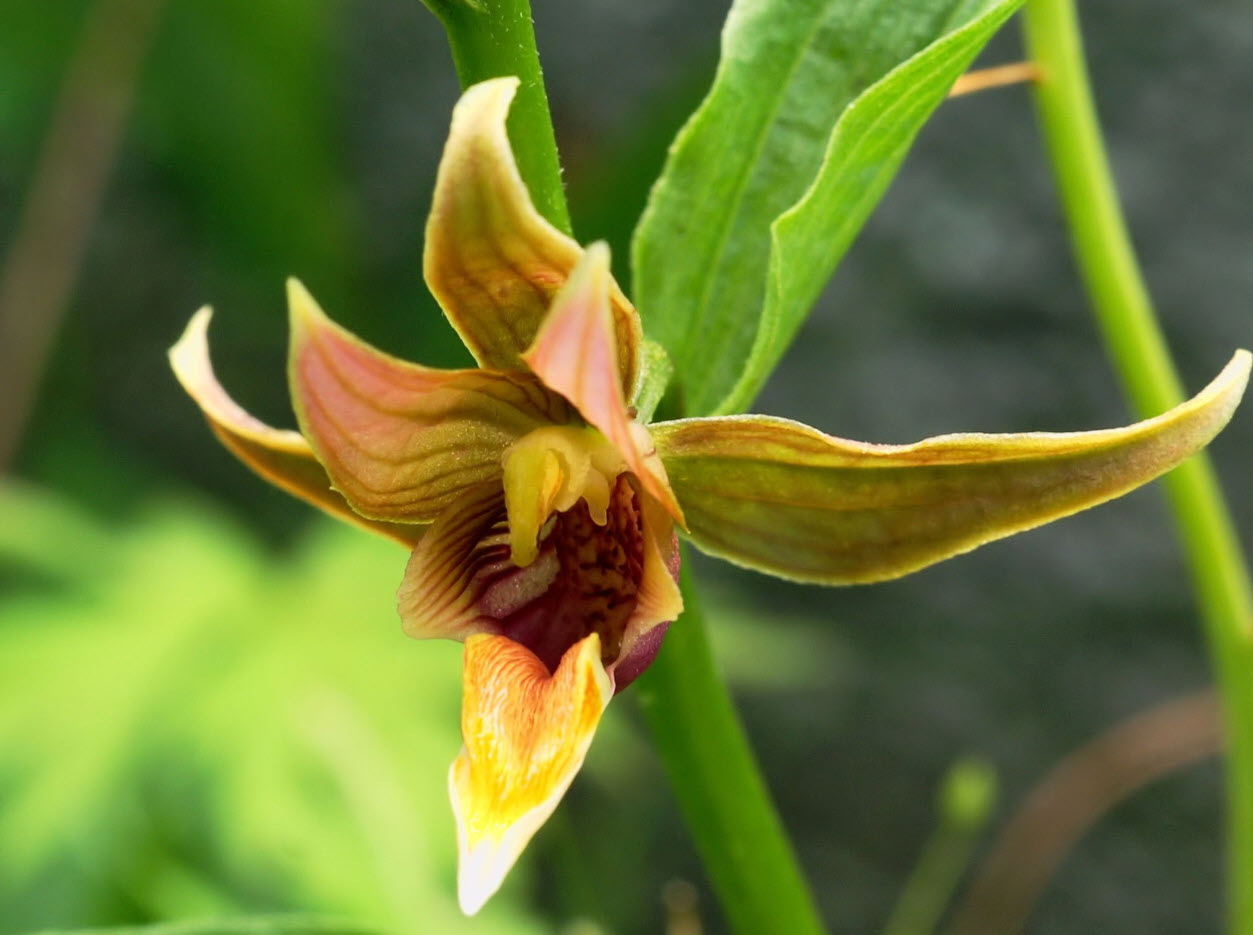This is a highly detailed close-up photo of a single bright yellow flower on a long, skinny green stem. The flower features a combination of colors: its predominantly yellow petals have brownish-green veins and pinkish-reddish tips. The center of the flower appears dark with red veins, adding to the intricate detailing. The petals, six in total, are triangular and slightly curved as if they are beginning to wilt. The background is very blurry, suggesting the presence of more green plants, and possibly a rocky shoreline, although these details are indistinct. There is another green stem visible but cut off before the flower, adding depth to the image taken in a natural, wild setting rather than a controlled environment like a vase.